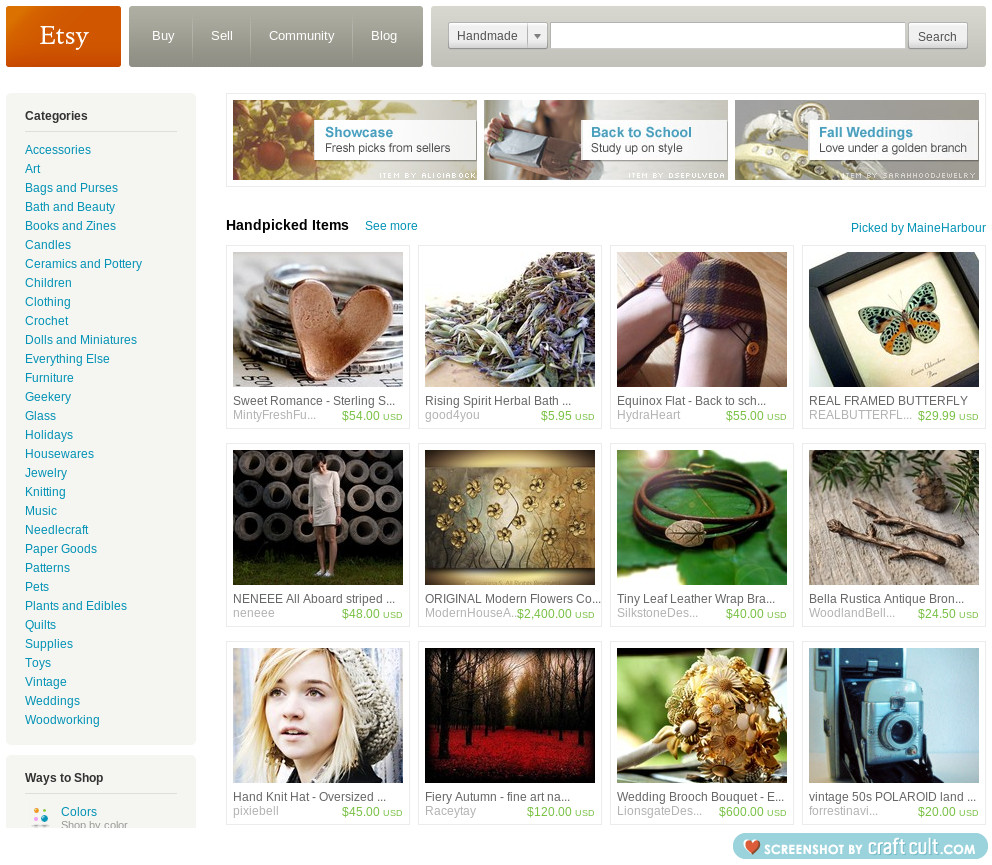This is a detailed screenshot of the Etsy website interface. 

At the top left corner, the Etsy logo is prominently displayed inside an orange box. Adjacent to it, within the same row, is a rectangular gray box featuring four links: Buy, Sell, Community, and Blog, listed horizontally. Following this is another rectangular box containing a search bar and a drop-down menu with "Handmade" as the first option. 

The main page has a clean, white background. On the left side, there is a vertical categories pane with more than 20 category links listed in blue text. The first three categories are Accessories, Art, and a subsequent category.

The right side of the page features a section titled "Hand-picked Items." This section showcases a grid layout with four pictures per row. Each image includes the item's price, written in green, a brief one-line description, and the seller's screen name. 

Highlighted prominently is the first photograph, which depicts a stack of silver rings topped with a copper heart, priced at $54.